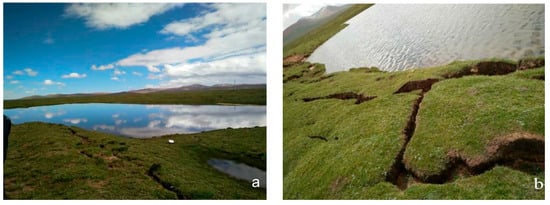The images consist of two stunning nature aerial photographs capturing serene landscapes featuring lush green terrain and tranquil lakes. 

In Image A, labeled with a small white "A" at the bottom right corner, the lake is surrounded by verdant, flat land. This photograph is taken from a flatter angle, showcasing the serene water that mirrors the blue sky and scattered clouds with impeccable clarity, creating a glass-like reflection. The sky above is partly clear with patches of clouds adding to the idyllic scenery.

Image B, marked with a small letter "B" at the bottom right, is shot from a more diagonal and downward angle. The lake, positioned towards the top right of the image, does not reflect the sky due to the water's visible ripples and movement. This gives the lake a slightly dynamic and textured appearance, contrasting with the smooth, reflective water in Image A. The green terrain occupies most of the photograph's foreground, enhancing the natural beauty of the scene.

Both photographs collectively highlight the contrasting states of the lake waters amidst a flourishing green landscape.